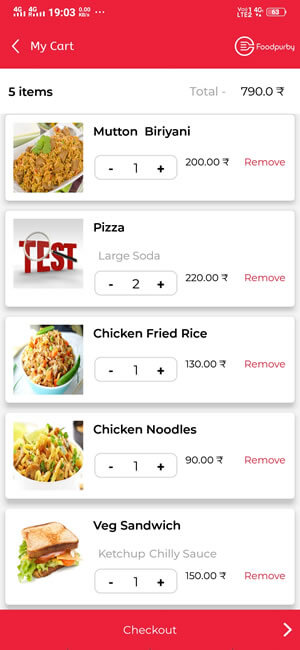The image depicts a mobile app interface for ordering food from the delivery service FoodPurby, identifiable by its logo and name in the upper left corner. The user's device is a dual SIM card phone, visible at the top right, showing two active 4G SIM cards with VoLTE functionality. The time indicated on the device is 19:03, using a 24-hour clock, suggesting an international setting, possibly in India, given the usage of the Indian Rupee.

The app screen displays the "My Cart" section, indicating that the user has added five items to their cart, totaling 790 rupees. The items listed include mutton, biryani, pizza, chicken fried rice, chicken noodles, and a vegetable sandwich, with prices ranging from 90 to 200 rupees each. Users have options to modify their orders by removing items or adjusting quantities. A checkout option is available at the bottom of the screen for finalizing the order. The phone's battery level is shown to be at approximately 63%.